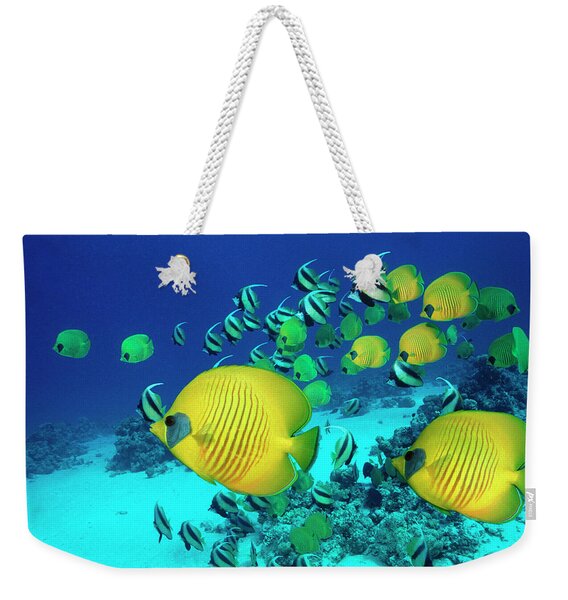The image features a highly detailed and almost surreal-looking tote bag with an underwater theme, against a plain white background. The tote bag is adorned with a realistic yet possibly computer-generated print of an ocean scene, highlighted by its pristine, perfect appearance. It has sturdy white rope handles for carrying. Dominating the foreground are two large yellow fish with black eyes, subtle green on their tails, and some gray around their eyes. Surrounding them are smaller yellow fish, including baby versions that could suggest a family, and a distinctive black and yellow fish with black stripes. The deeper parts of the scene reveal an ocean floor that’s white and sandy, dotted with coral and accented by various shades of blue from light to deep. There's a scattered presence of more marine life, including little pink creatures that might be jellyfish. The entire image evokes the hazy, illuminated look of the deep ocean, making this beach-ready tote bag both vibrant and spacious, ideal for carrying a lot of items.